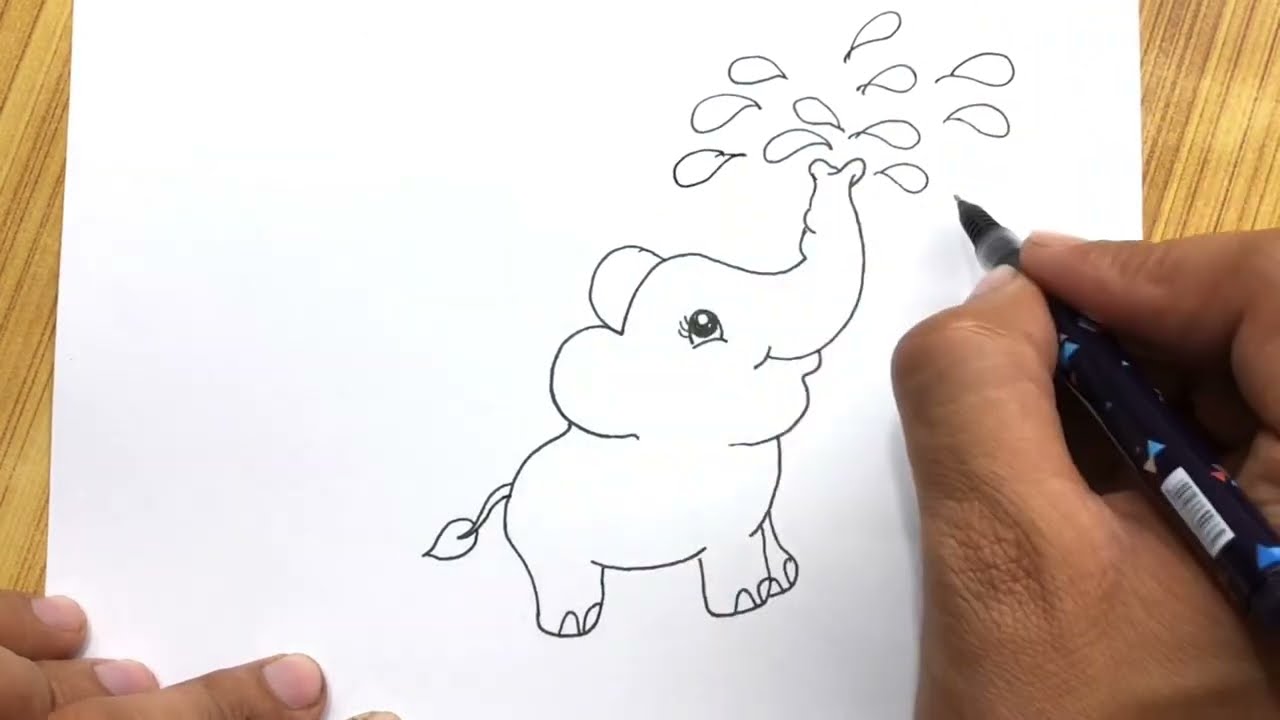The image depicts a color photograph in landscape orientation, showcasing a person's hands as they draw an illustration on a white piece of paper. The setting includes a woodgrain tabletop beneath the paper. In the bottom right-hand corner, the right hand, holding a pen that resembles a Sharpie, actively draws an outline of a playful baby elephant. The left hand, with fingers—including some with dirty fingernails—rests at the bottom left corner, holding the paper in place. The black ink drawing features a cartoon-like baby elephant with large eyes, long eyelashes, and a tail with a fig leaf at the end. Its trunk is raised and appears to be spraying drops of water, depicted in a simple, black line art style. The overall scene is one of photographic representationalism, highlighting the process of creating this charming illustration.